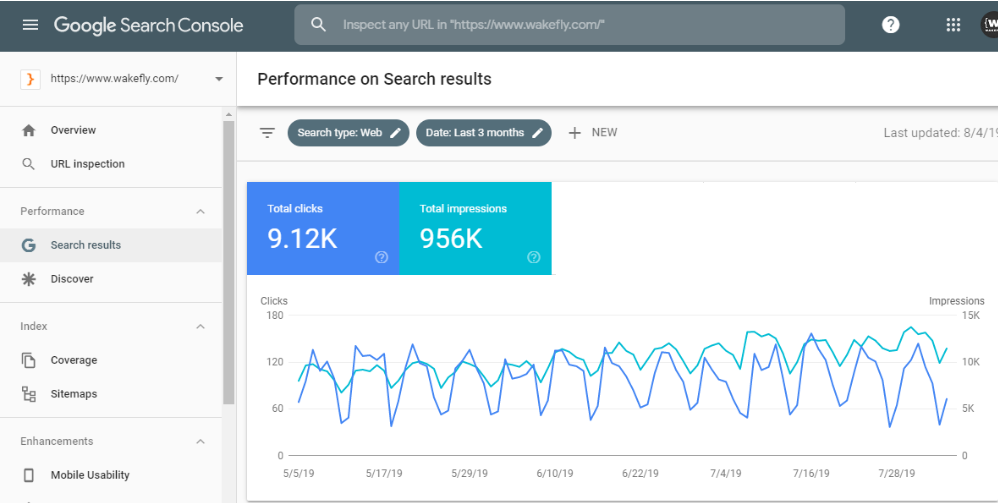The image showcases a detailed interface of the Google Search Console dashboard. 

At the top, there's a blue-gray header with a menu icon featuring three horizontal lines on the left. Adjacent to the icon, the text "Google Search Console" is clearly visible. Within this header is a lighter gray search bar containing a magnifying glass icon and some unreadable white text. To the right of the search bar, there's a white circle with a question mark inside, followed by a grid of dots symbolizing a settings or options menu. At the far end of this header is a truncated icon that seemingly contains a "W" character.

Below the header, the next section has a white background featuring a right-pointing arrow accompanied by some text. Here, it also reads “Performance on search results.”

On the left sidebar, starting from the top, there is a small home icon labeled “Overview”, followed by an icon of a magnifying glass labeled “URL Inspection,” and another section labeled “Performance” with an upward-pointing arrow next to it. Further down, a green-gray "G" icon represents “Search Results,” and a starburst icon signifies the “Discover” section. There's also a folder-like icon labeled “Index,” within which “Coverage” is specified next to an icon resembling two overlaying sheets of paper, and an unreadable symbol possibly related to enhancements.

Directly under the “Performance on search results” heading, there's a gray line. Below this, a segment indicates "Search type: Web" featuring a blue-gray Wi-Fi-shaped icon, and "Date: Last 3 months" with a corresponding line. A gray plus sign labeled “New” is present, followed by the text “Last updated: 8-4,” although this information is partially cut off.

On the right side, there's a blue bar with some unreadable white text. It displays the number "9.12k" alongside a small symbol at its lower right. Beneath this, a light blue-green bar contains more unreadable text showing "9.56k" with a small symbol at its base.

At the bottom of the image, a chart visualizes data with lines colored in similar blue and blue-green shades from the aforementioned bars. This chart includes numerical annotations along both the vertical and horizontal axes, representing performance metrics over time.